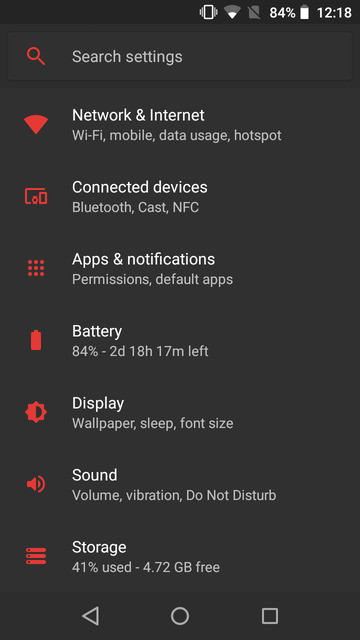The image depicts a cell phone screen displaying the Settings menu. The battery icon at the top right shows 84% power remaining, with a time indication of 12:18. A mix of familiar and unfamiliar icons are present. Dominating the black background, all icons are highlighted in red and general text appears mainly in white and gray. The initial text, "Search Settings," is in gray, followed by menus such as "Network & Internet," where further options are listed as Wi-Fi, mobile data usage, and hotspot. Underneath, the "Connected Devices" section features Bluetooth, Cast, and NFC settings. The "Apps & Notifications" section follows, detailing permissions and default applications. The battery details show 84% with an estimated lifespan of two days, 18 hours, and 17 minutes left. Additional categories include "Display" (wallpaper, sleep, font size), "Sound" (volume, vibration, Do Not Disturb), and "Storage," which indicates 41% used with 4.72 GB free. At the bottom of the screen are navigation icons: a left-facing arrow for 'back,' a circle for 'home,' and a square for 'recent apps,' all outlined in white. The specific unidentified icon described is a square with progressively smaller bars on either side, possibly signifying a signal or data-related function.